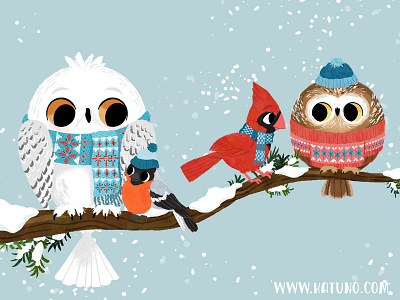This charming illustration from www.katuno.com depicts a whimsical winter scene with a light blue, snow-adorned background. Four colorful birds sit cozily on a snow-dusted tree branch with scattered green leaves. On the far left, a white owl with big black eyes, highlighted by a beige color, sports a festive blue scarf decorated with red holly. Beside the owl, a small creature, likely a mouse, wears a two-tone blue knit hat and a bright orange sweater. A vibrant red cardinal, donning a blue holiday scarf, perches next to the mouse. Completing the scene on the far right, a brown owl is snug in a red knitted sweater with festive designs and a matching two-tone blue hat. The entire image exudes a warm, holiday spirit, perfect for a Christmas card.